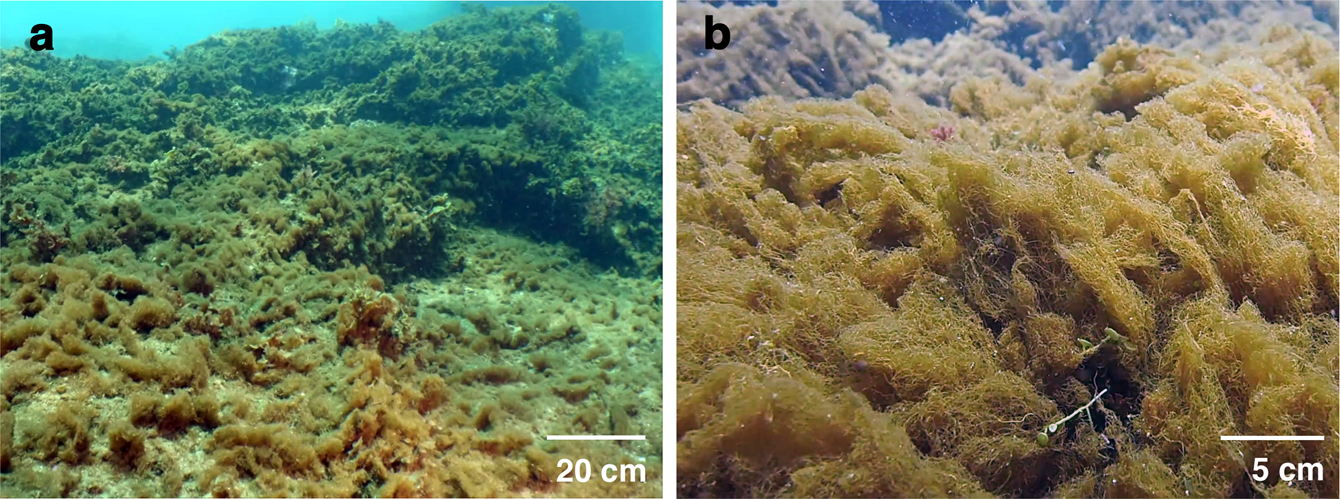The image is a composite of two side-by-side, underwater landscape photographs, separated by a vertical white line. The left photograph is labeled with a lowercase 'a' in the top left corner and includes a scale marker of 20 centimeters in white text at the bottom right corner. The right photograph is labeled with a lowercase 'b' in the top left corner, with a scale marker of 5 centimeters in the bottom right corner. Both images feature underwater scenes likely intended for scientific analysis, potentially for a textbook or journal paper.

In image 'A,' the seafloor is depicted with a variety of elements: predominantly rocky and hard coral structures with a mixture of dark gray and black tones in the shadowed areas. There are patches of green algae and some sparse orange, spongy material, which may indicate the initial stages of erosion or colonization by sponges. The broader scale of 20 centimeters suggests a more extensive view of the seafloor composition.

Image 'B,' on the right, is a closer view, depicted at a 5-centimeter scale, focusing predominantly on a brown, sponge-like material. This material exhibits a fibrous, undulating surface with numerous ridges and potentially illustrates a more detailed look at the sponge colonization process or the effects of erosion over time. The predominance of the spongy texture emphasizes the biological interactions occurring on the ocean floor, and the presence of some orange spongy material links it visually to the content in image 'A.'

Both images serve as complementary views of the underwater environment, showing different scales and levels of detail in the seafloor's biological and geological features.